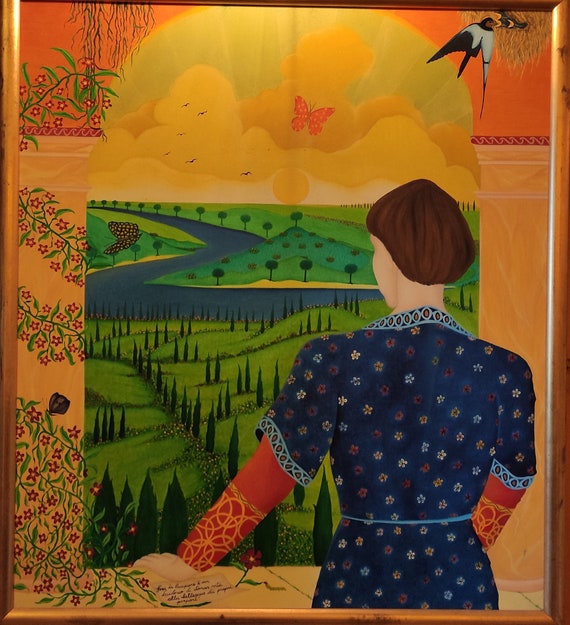The painting depicts a woman in a blue dress adorned with floral designs, complemented by a red long-sleeved shirt underneath. Her attire features golden intersecting rings around the cuffs and forearm area. She has short brown hair, and her back is turned to the viewer, as she gazes out through an arched window with an orange border. The window frame is entwined with a winding vine that climbs up the left side. 

In the background, a serene valley unfolds with a winding river flowing through verdant hills and neatly cared-for trees. The sky above is yellow, punctuated by white and yellow clouds, with a bright orange butterfly speckled in the center. In the upper right corner, a bird is seen feeding its chicks in a nest. The detailed craftsmanship of the golden frame encasing the artwork adds a touch of elegance to the entire scene.